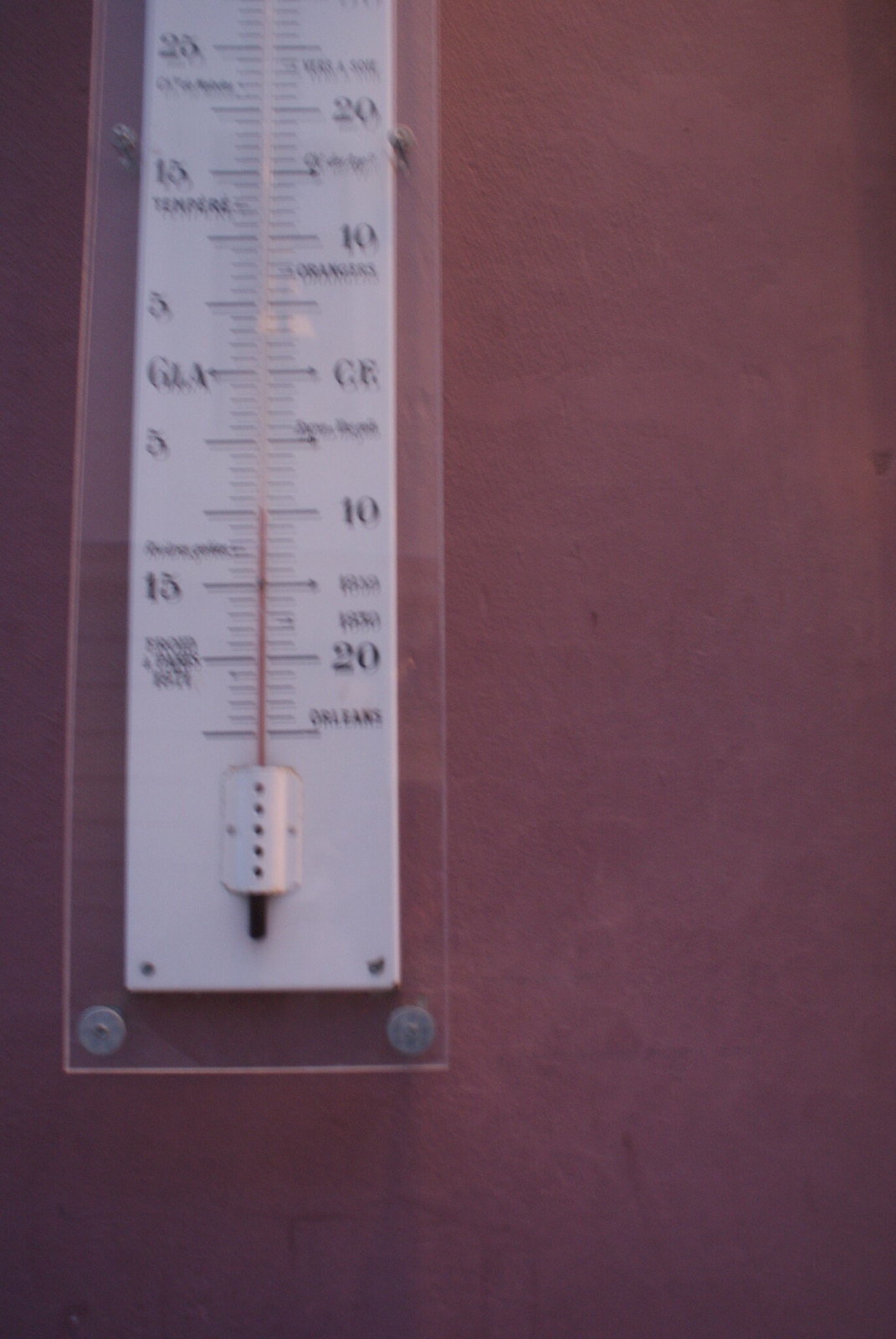The image depicts a dark purple background, likely a wall, with a temperature gauge mounted on it. The gauge is partially visible, revealing only the bottom portion. The gauge has numeric values on its sides – '25' on the left and '20' on the right. The precise language of the text inscribed on the gauge is indiscernible, but black lettering on a white background is noticeable. The thermometer itself contains red ink indicating the temperature, and it is secured with a white, screwed clamp attached to the thermometer's plate. The current temperature reading hovers around '10' on the right side, though the image is slightly out of focus, making it challenging to clearly identify the gauge type or its exact reading.